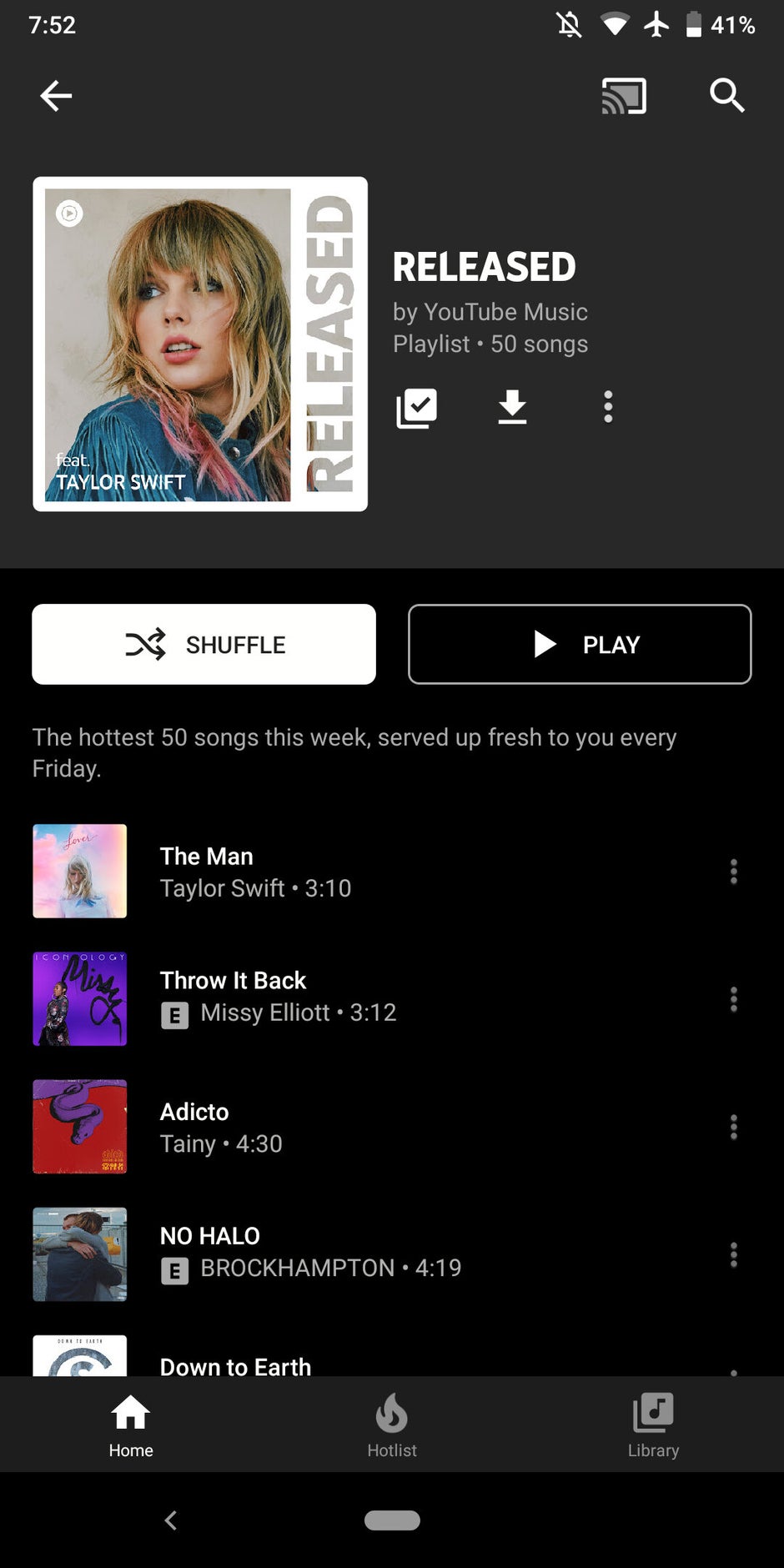The image shows a screenshot of a mobile device at 7:52 AM, as indicated in the top-left corner. In the top-right corner, icons for mute, Wi-Fi, airplane mode, and a battery level at 41% are visible. Below, a navigation bar with a back button, "Taylor Swift" released by YouTube Music, and playlist details which include 50 songs, shuffle, and play options. The visible tracks are "The Man" by Taylor Swift (3:10), "Throw It Back" by Missy Elliott (3:12), "Addicto" by Tini (4:30), and "No Halo" by Brockhampton (4:19). Further down, menu options for Home, Hotlist, and Library are displayed along with an additional back button and navigation pill.